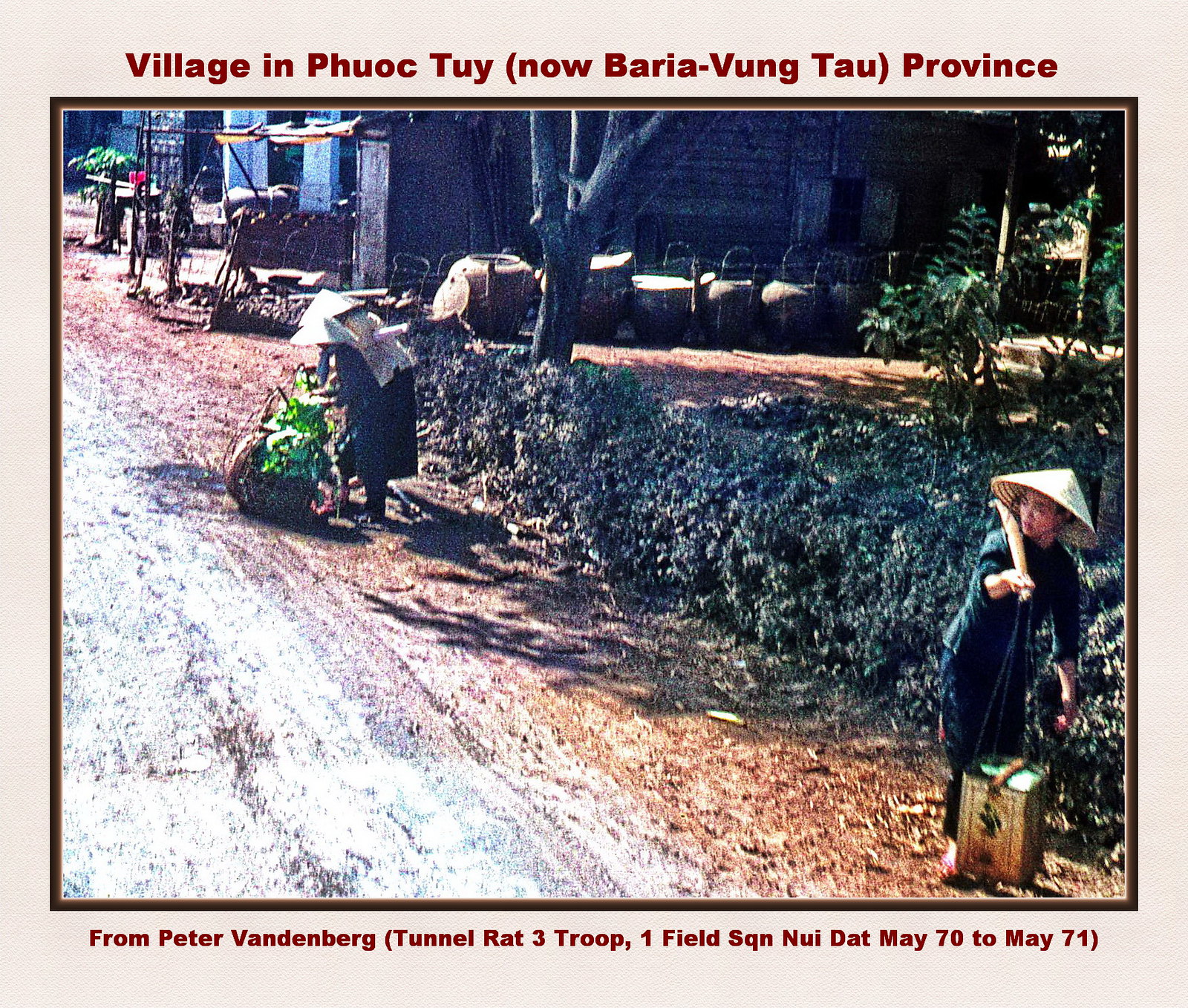This image captures a nostalgic scene from Vietnam, specifically a village in Phuoc Thuy, now part of Vung Tau Province. The photograph, taken by Peter Vandenberg of Tunnel Rat 3 Troop, 1 Field SQN, during his service from May 1970 to May 1971, showcases a serene midday moment with two Vietnamese women engaged in their daily labor. Both women are dressed in traditional Vietnamese garments, with one donning the iconic conical hat. The woman in the bottom right corner is seen carrying a pail of water in a box-like carrier, while the woman toward the top left-hand side is handling bundles of plants, leaves, and wicker baskets. They stand along a road flanked by lush grass, trees, and bushes, with simple houses or shacks in the background. The image is rendered in muted tones of gray, green, beige, brown, blue, red, and tan, capturing the earthy essence of rural Vietnam. Text overlays at the top and bottom of the square photograph provide context and provenance.